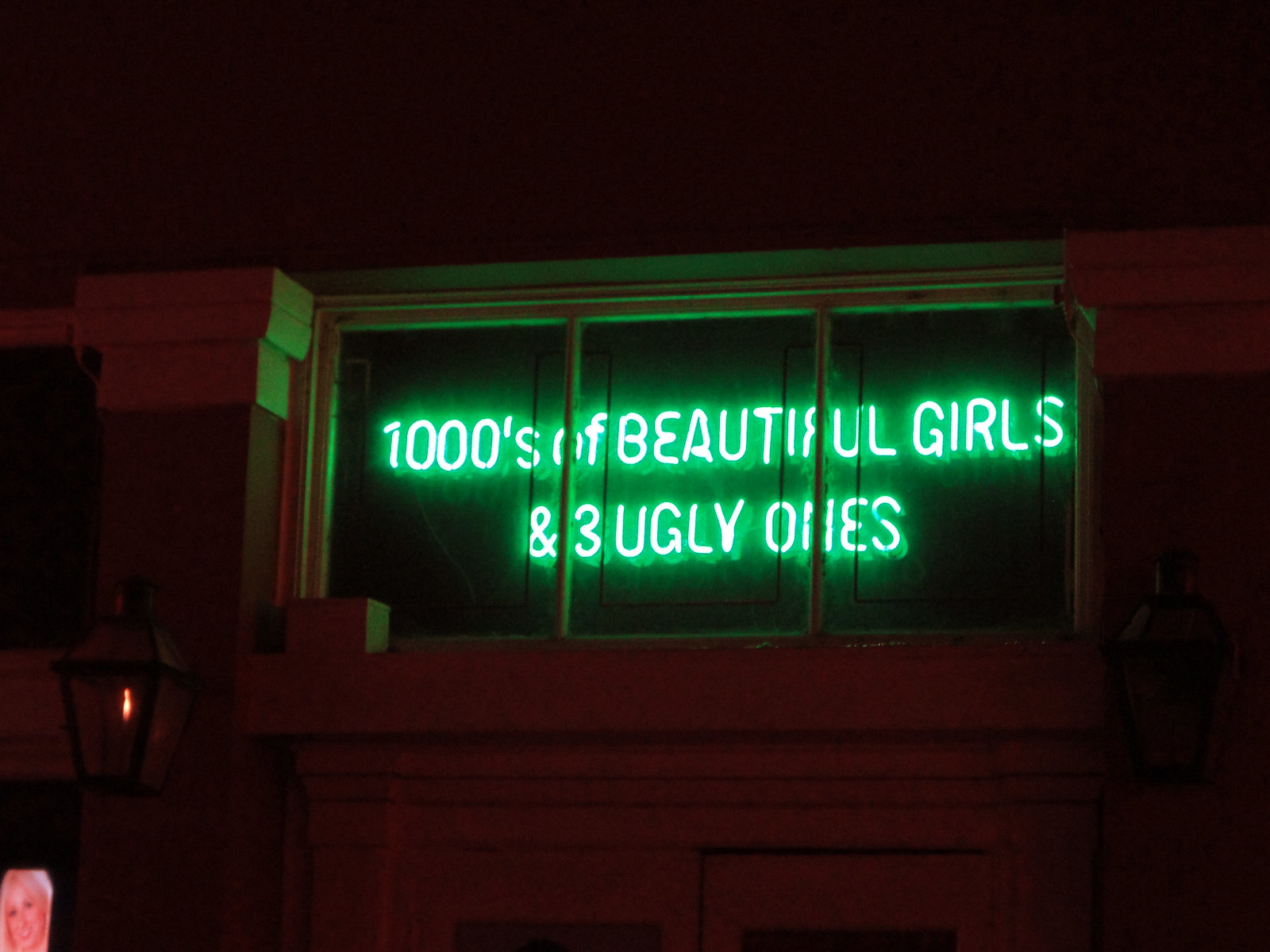The image depicts an outdoor night scene featuring a dimly lit building with a classical architectural style, characterized by concrete material and columns. The building's exterior includes a rustic, gaslight-style streetlight affixed to its left side, emitting a modest glow. A prominent window, divided into three vertical panes, is situated high up on the wall and houses a striking neon green sign. This sign boldly declares, "Thousands of beautiful girls and three ugly ones," suggesting the building may be a club or strip club. Although the structure's precise colors are hard to discern due to the poor lighting, hints of darker red and lighter beige are visible. In the bottom left corner, partially obscured and likely seen through a doorway, is the projected image of a blonde woman with long hair.